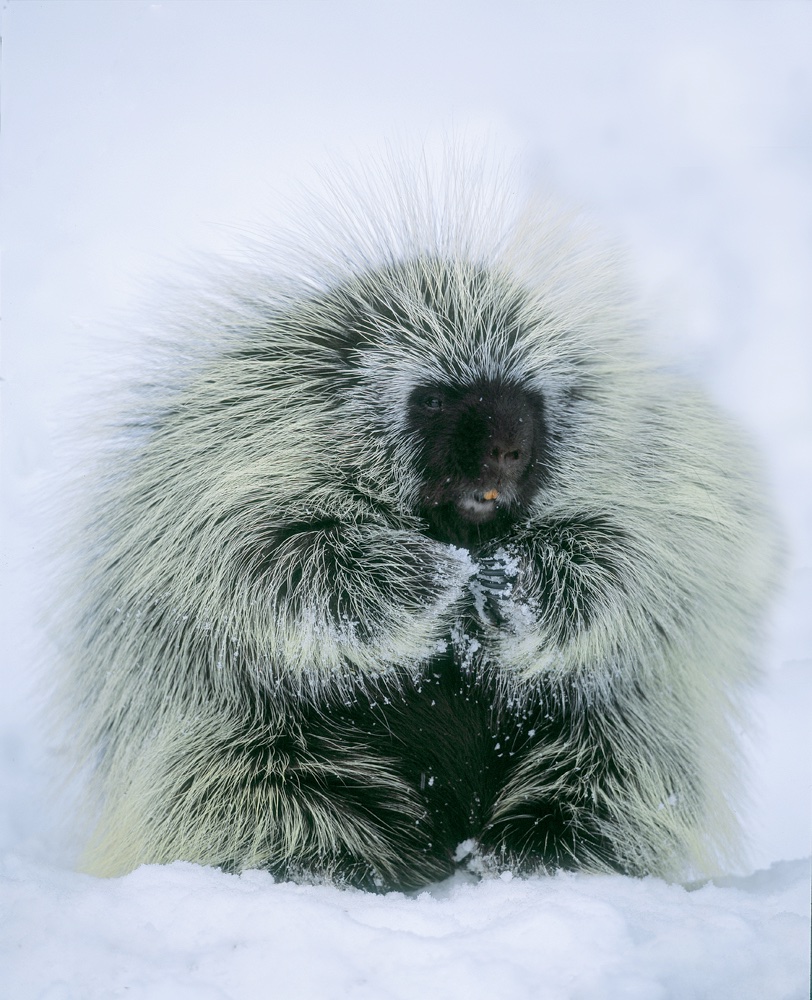This vertically aligned, rectangular close-up image showcases a peculiar animal blending traits of both a porcupine and a bear. It features a dark brown face, almost black, reminiscent of a baby bear or an ape, with small black beady eyes and something orange dangling from its mouth. The creature's body is enveloped in a luxurious coat of long, white, spiky fur, akin to porcupine quills or an extravagant fur coat. Its arms and back are similarly covered, with hints of snow and ice clinging to the fur, indicating it is sitting on a snow-covered ground. The background of the image is a serene blur of white, suggesting a snowy environment or possibly a white sky. The animal appears to be huddling, perhaps for warmth, and stares directly at the camera, creating a striking contrast between its dark face and the bright, spiky fur that encases its body.